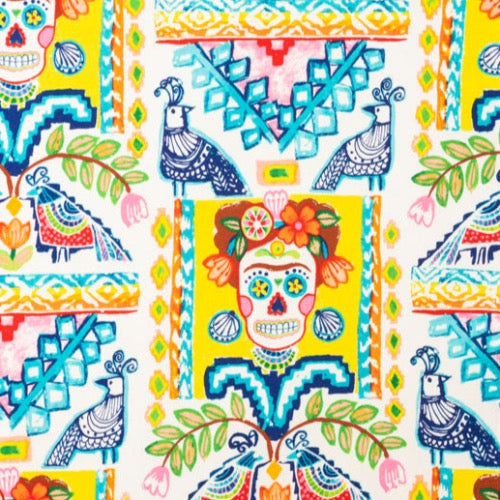The square image captures a vivid, high-contrast design reminiscent of a tile or fabric pattern, bursting with vibrant colors like blues, yellows, pinks, reds, and oranges. At the heart of the image lies a Dia de los Muertos-inspired sugar skull set against a bright yellow background. This cheerful, cartoonish skull features prominent red hair adorned with colorful flowers and fruits, a unibrow, and large, expressive teeth. Shell earrings dangle from where its ears would be, adding a touch of whimsy. The skull's eyes are depicted as flowers, enhancing its festive appearance. Surrounding the central skull are intricate designs, including geometric motifs and repeating prints of blue peacocks—four of them prominently placed in the corners. Interspersed among these elements are green and yellow leaves emerging from stems, culminating in pink flowers. The entire composition forms an elaborate and harmonious pattern, evoking the rich tapestry of Mexican cultural art.